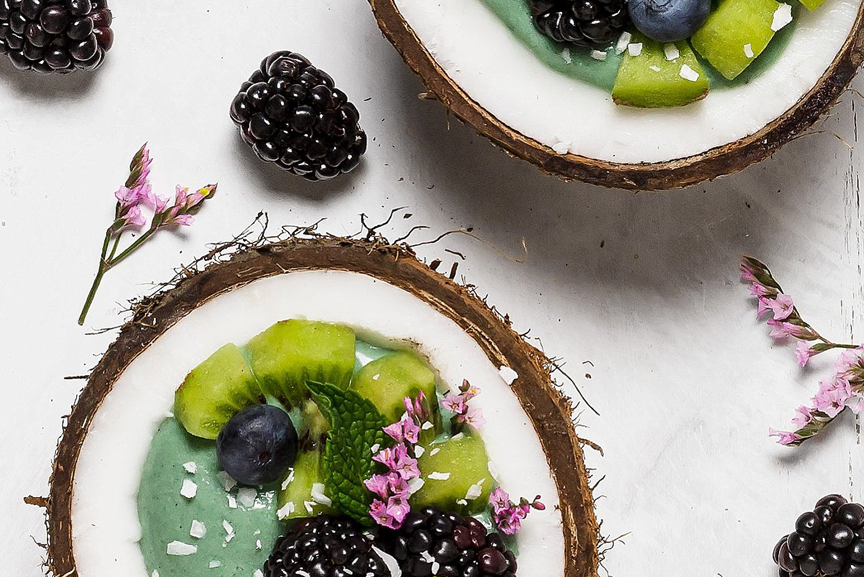In this visually captivating image, a white table serves as the background, scattered with several plump blackberries displaying their deep, dark hues with white reflections. The centerpiece of the composition features two artistically arranged plates resembling cut-open coconuts, their rugged brown exteriors contrasting with the smooth white interiors. Each plate contains an exquisite assortment of fruits including vibrant green melon slices, succulent kiwifruit, a single blueberry, and more blackberries. The presentation is further enhanced by the inclusion of mint leaves, adding a fresh pop of green. Small, delicate dried pink flowers are interspersed among the fruits, lending a touch of whimsical elegance. Additionally, a green jelly-like substance, possibly pistachio ice cream, shares space with the fruits in these unique coconut-shell plates. A plum and a couple of these charming purple flowers lie nearby, adding further color and detail to this intricate and aesthetically pleasing arrangement.